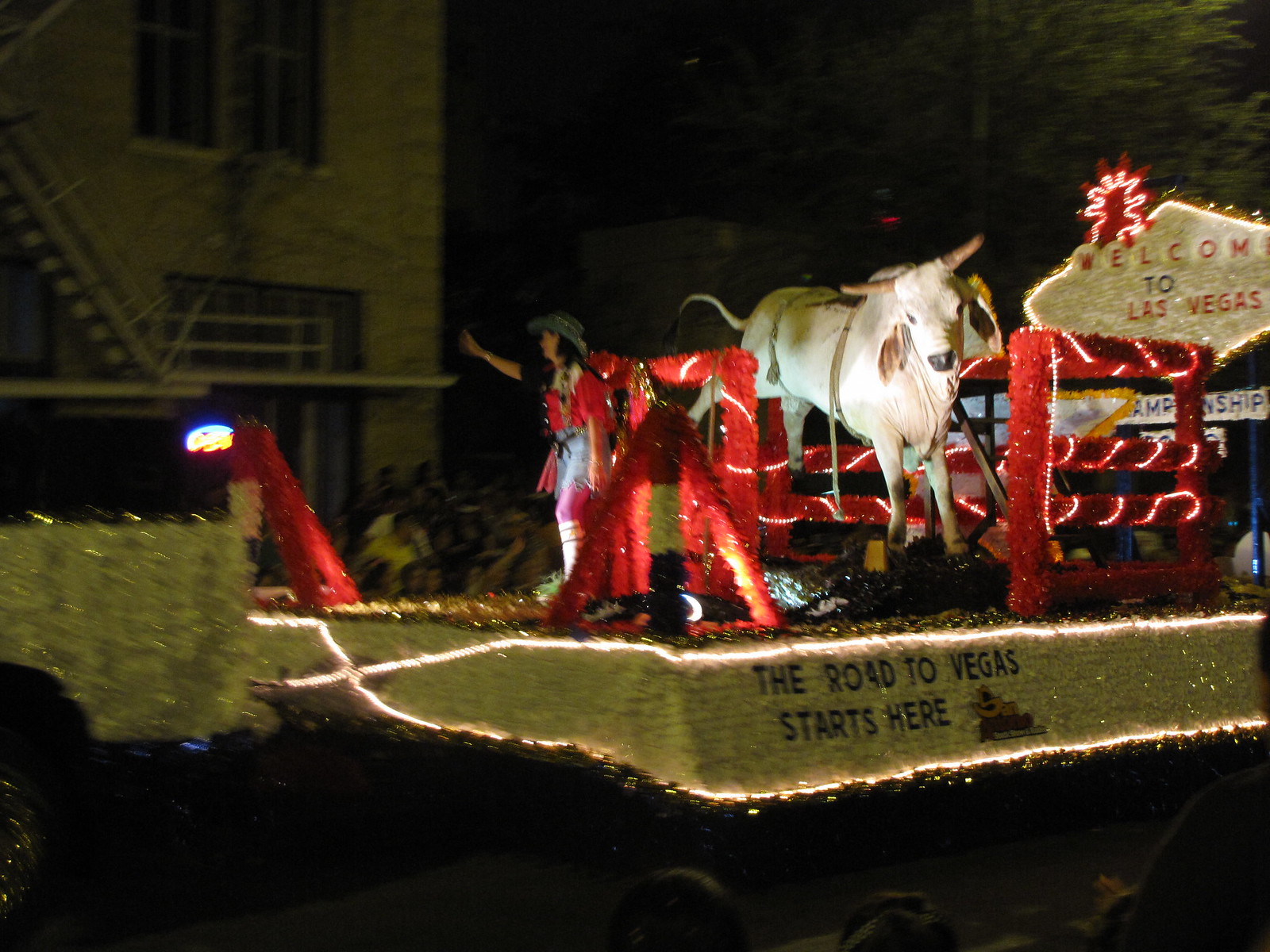The image captures a vibrant nighttime parade float with an elaborate gold sparkly base adorned with lights. Dominating the float is a corral area accentuated by a red decorated gate. Inside the corral stands a beige longhorn bull, clearly a prop, surrounded by a glittery fence. A lady commands attention at the front of the float, dressed in a sparkling cowgirl outfit complete with a cowboy hat, high boots, blue jeans, and a shirt. She waves energetically to the crowd gathered along the parade route. Behind her, a lit-up gold sign mimics the sparkle of the float and reads "Welcome to Las Vegas," reinforcing the float's lively theme. Additional text on the float's base declares, "The road to Vegas starts here." In the background, blurred buildings and a truck towing the float frame the scene, hinting at the festive atmosphere with people waving and enjoying the special event. The image is a riot of colors, featuring hues of red, gold, black, white, gray, off-white, blue, yellow, brown, peach, and pink. Overall, the scene is festive and visually engaging, capturing the essence of a celebratory parade heading towards Las Vegas.